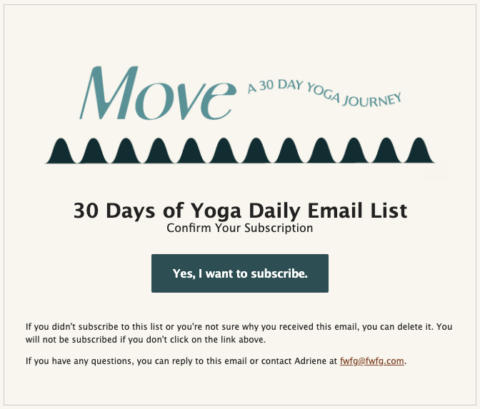The image features a promotional message from a yoga subscription service. It highlights a "30-Day Yoga Journey" program that entails daily email updates for 30 days of yoga practices. The text prominently encourages the reader to confirm their subscription by clicking a link with the phrase "Yes, I want to subscribe." Additionally, it reassures the recipient that no action is needed if they did not intend to subscribe or are unsure why they received the email. The message also notes that the recipient will not be subscribed unless the link is clicked. For any questions or concerns, recipients are instructed to respond to the email or contact Adrienne at fwfg@fwfg.com. The overall design is clean and informative, guiding users through the subscription process clearly.